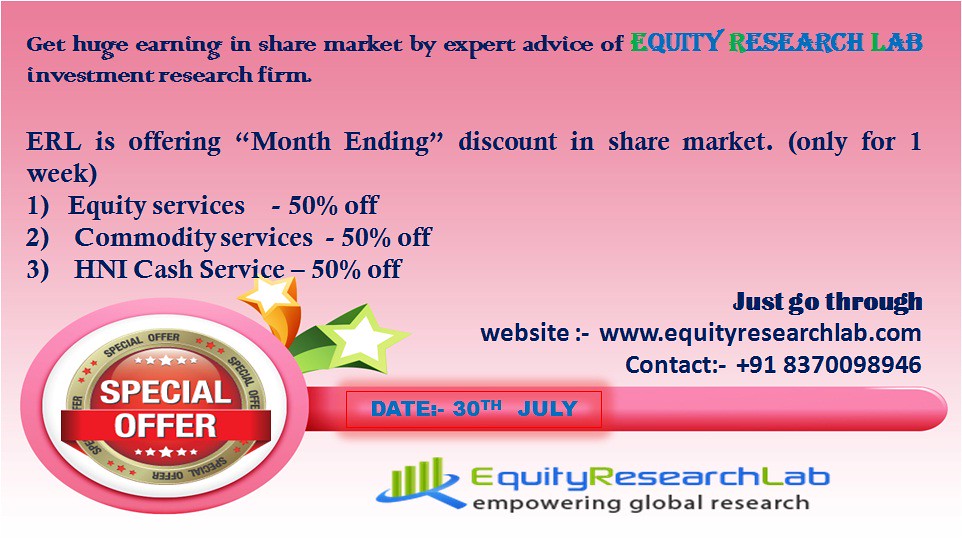The advertisement features a horizontally aligned rectangular image with a gradient background that transitions from dark pink at the top, through light pink, and into white at the bottom. 

At the top left, in dark blue print, the main headline reads: "Get huge earning in share market by expert advice of Equity Research Lab, investment research firm." The words "Equity Research Lab" are prominently displayed in all caps, where the letters "E," "R," and "L" are green, and the remaining letters are bright blue. 

Beneath this, aligned to the left, it states: "ERL is offering month-ending discount in share market (only for one week)." Following this announcement, three offers are listed:
1. Equity services - 50% off
2. Commodity services - 50% off
3. HNI cash service - 50% off

On the lower left corner, there is a visually striking circular badge shaded in red with large white text reading "Special Offer." This badge is adorned with a row of white stars above the word "Special" and another star below "Offer," both of which are outlined in gold.

To the right of the badge, set against a bright pink background, the date "30th July" appears in blue text. Positioned just above this date, it boldly states "Just go through" in black text. Beneath this, the website "www.equityresearchlab.com" and contact number "+918370098946" are listed. 

At the very bottom, centered, is the logo of Equity Research Lab which is colored in green and blue. It reads "Equity Research Lab, empowering global research," with the letters "E," "R," and "L" in green and the rest in blue.